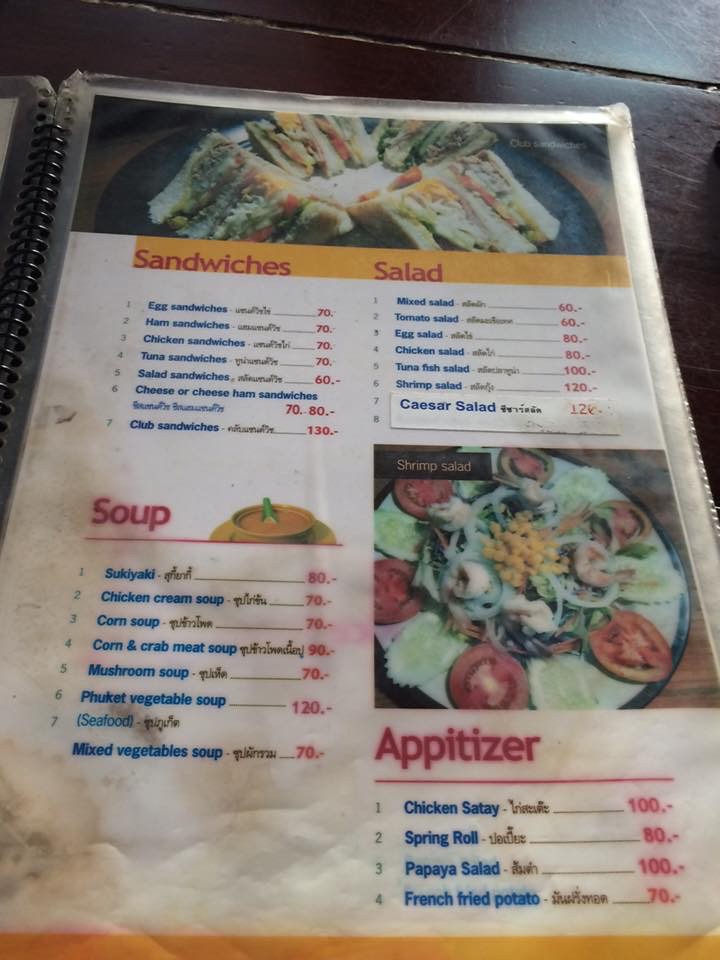This photograph captures a close-up view of a dark brown wooden table with an open menu laid out across it. The menu, encased in a clear plastic cover, features a series of black spring bindings on the left side for secure page turning. At the top of the right-hand page, a vibrant image of a sandwich is prominently displayed, leading into a section labeled "Sandwich, Salad" in bold red text.

The listed sandwich options include:
- Egg Sandwich
- Ham Sandwich
- Chicken Sandwich
- Tuna Sandwich
- Salad Sandwich
- Cheese or Cheese Ham Sandwich
- Club Sandwich

Each sandwich is accompanied by its price, clearly marked in red.

Below, the menu transitions into various salad options, also listed with their prices in red:
- Mixed Salad
- Egg Salad
- Chicken Salad
- Tuna Fish Salad
- Shrimp Salad
- Seeds Salad

Further down, a red heading announces the "Soup" section, featuring an array of soup choices with corresponding prices in red:
- Chicken Cream Soup
- Corn Soup
- Corn and Crab Soup
- Mushroom Soup
- Vegetable Soup
- Mixed Vegetable Soup

A detailed picture of a shrimp salad adds a visual appeal, positioned just above the "Appetizer" section, indicated in red text. Listed appetizers include:
- Chicken
- Spring Roll
- Papaya Salad
- French Fried Potatoes

These are also presented with their respective prices in red, completing the detailed and well-structured layout of the menu.